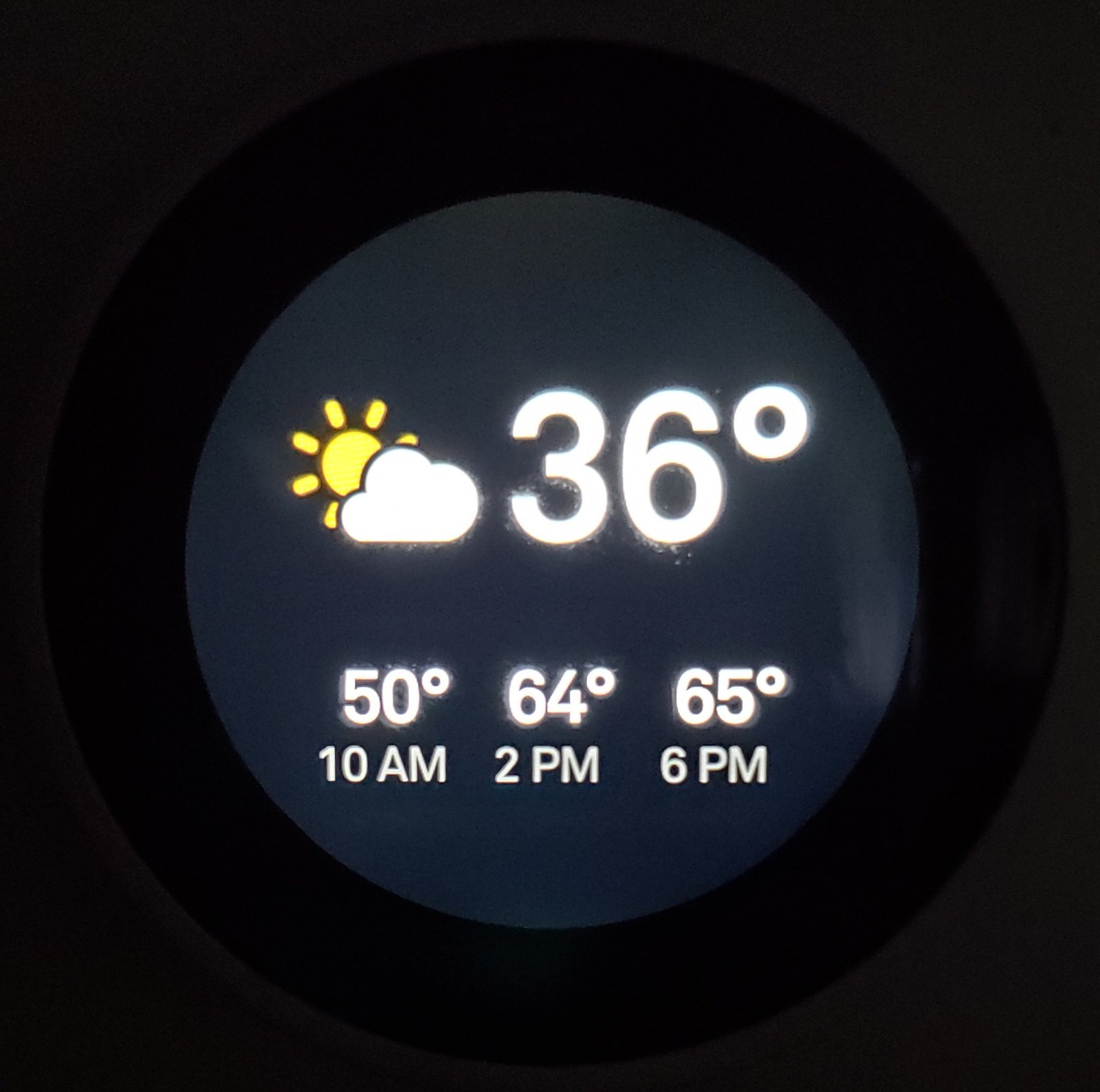This image features a predominantly dark background, almost approaching a grayish tone. Dominating the center is a thick, black circle set against a dark gray backdrop. Towards the right side of the circle, a small white smudge is noticeable. At the top of the circle, a white cloud is depicted, accompanied by a yellow circle representing the sun, which has splatters or spots extending from it.

To the right of this graphical composition, large white text displays "36°." Directly below, "50°" appears in white letters. Continuing downward, the text "10 a.m." is shown. Adjacent to this, more text in white reads "64°," and beneath it, "2 p.m." Finally, towards the bottom right, the text "65°" is displayed above "6 p.m." This comprehensive arrangement of text and graphics likely provides weather details over specific timestamps.